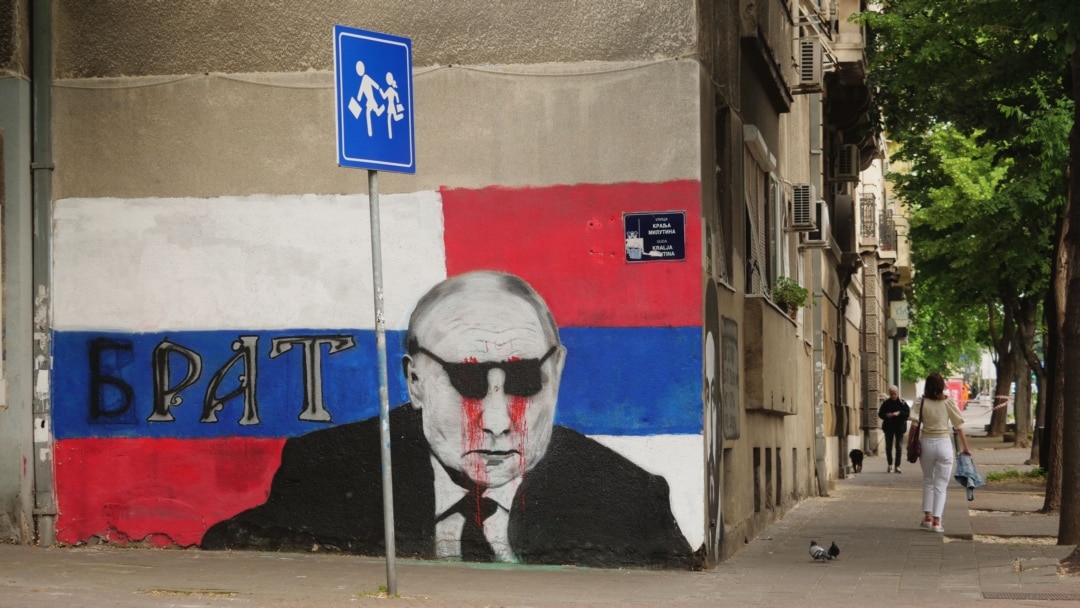The photograph captures a bright and clear urban street corner. Dominating the scene is a beige building adorned with graffiti art. The graffiti features a vivid depiction of Vladimir Putin wearing black sunglasses, with red blood graphically streaming from both his eyes and down his face. The artwork is detailed with a black square in the top right corner, and a blue line through the center bearing the letters "B.P.A.T." Near his shoulder, a red and white stripe is prominently visible.

On the right side of the street, trees with lush green leaves frame the sidewalk filled with activity. A woman dressed in white pants, a yellow short-sleeved shirt, and white shoes walks away from the camera. Nearby, an older person with white hair in an all-black outfit walks a dog towards her. Two pigeons are also seen at the street corner. A blue street sign featuring children running and a red, white, and blue flag add splashes of color to the busy setting, further emphasizing the urban life captured in this moment.